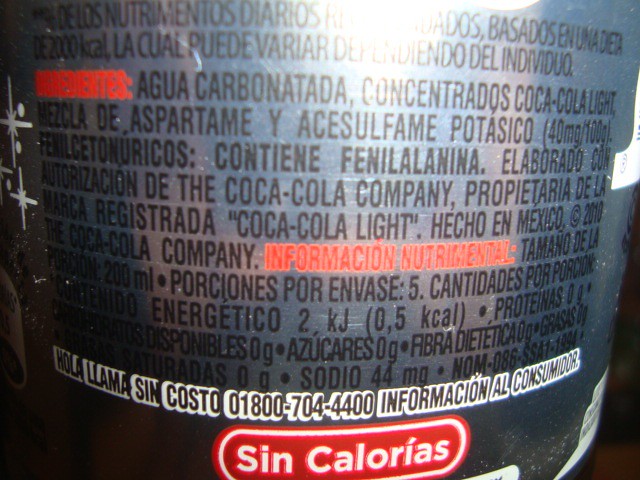This photograph showcases the list of ingredients on the back of a round, silver Coca-Cola Light can. The can features black lettering with sections reflecting light, making parts of the text challenging to discern. 

Prominent at the bottom is the phrase “sin calorías,” Spanish for "zero calories," affirming the drink's lack of caloric content. The detailed nutritional information is partially visible, indicating that the beverage contains no calories, carbohydrates, or proteins, aligning with diet standards that may vary between individuals.

Key ingredients are listed in Spanish: "agua carbonatada" (carbonated water) and "concentrados de Coca-Cola Light" (Coca-Cola Light concentrates). The can also mentions the presence of "aspartame" and "acesulfame potassium" at 40 milligrams. There's a caution about the presence of "fenilalanina" (phenylalanine), essential for those with certain dietary restrictions.

The light's glare obscures some parts of the text, while the darker bottom segment of the can makes it harder to read. Despite this, the clean labeling in Spanish provides a clear indication of the contents and dietary information of this Coca-Cola variant.